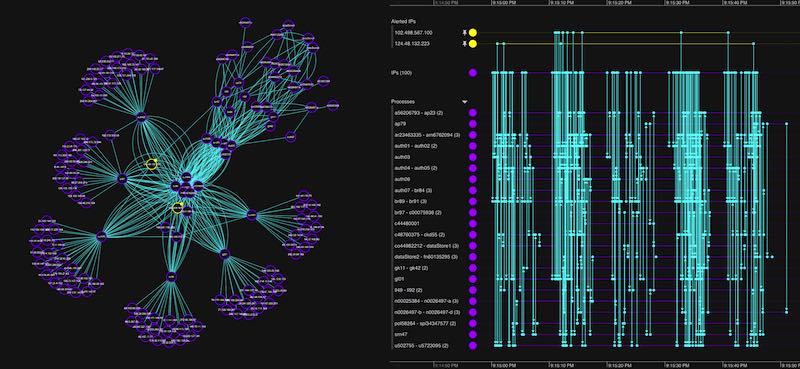The image is a detailed scientific visualization, likely depicting DNA strands and associated data. The left side features a molecular diagram consisting of several bowed teal lines bundled together at points resembling hairbands, with purple circles at the tips. Two specific points within this diagram are highlighted in yellow. The right side presents what appears to be a graph, structured with rows of names marked by purple dots. Additionally, this section includes vertical teal bars that may indicate various measurements or data values. The entire image is displayed on a computer screen, approximately two and a half times wider than it is tall, combining graphical and textual elements to convey complex scientific information.